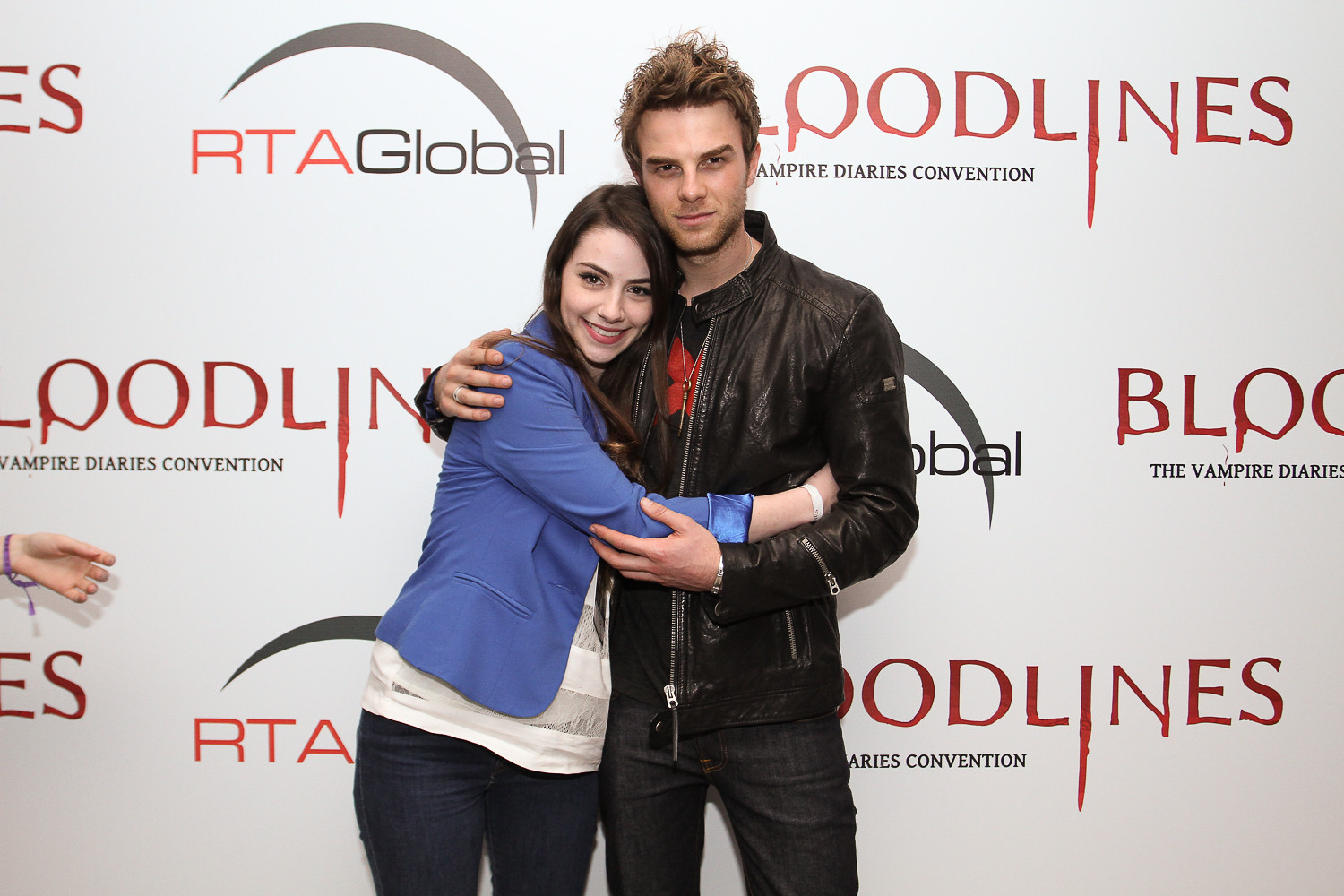In this vibrant image, a young couple in their early 20s stands affectionately in front of a large white billboard filled with various advertisements, prominently featuring "Bloodlines" in bold red letters and "Vampire Diaries Convention" in black text. The man, positioned to the right, has short, messy light brown hair with darker undertones and sports an afternoon shadow. His black leather jacket, detailed with zippers, partially covers a black T-shirt adorned with a red symbol. Black jeans complete his edgy outfit. He dons a serious expression, with squinting eyes, as he wraps his right arm around the woman’s shoulder and his left hand under her right elbow. The woman, standing slightly to his left and facing the camera with a bright smile, has long, straight brown hair flowing down her back. She wears a blue jacket over a white and gray shirt, paired with dark jeans. One of her arms encircles the man's waist while the other is draped across his back. Her head is nestled against his neck, exuding warmth and closeness. Intricate elements of the billboard, such as the intertwined "RTA Global" text with a crescent moon, form a patterned backdrop, reinforcing the scene's thematic ties.